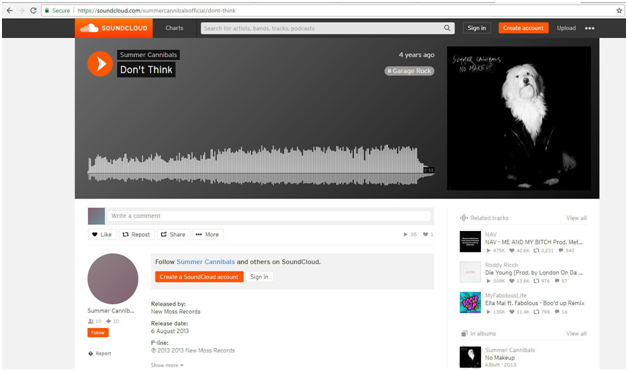The image features a user interface against a gray background, primarily concentrated in the top left area. A sequence of three arrows are displayed: a gray arrow pointing left, followed by a very light gray arrow pointing right, and a gray curved arrow indicative of a refresh icon. Adjacent to this is the word "secure" in green text, accompanied by a hyperlink to SoundCloud (soundcloud.com).

Below this, a prominent orange button labeled "SoundCloud" in white text includes a SoundCloud logo to its left. Next to this button is the word "Charts" in gray text. Positioned below these elements is a search box with placeholder text that reads, "Search for artists, bands, tracks, podcasts," paired with a magnifying glass icon symbolizing search functionality.

To the right of the search box, there are three buttons for user interaction: "Sign In" rendered in white text, "Create Account" on an orange button with white text, and "Upload" also in white text. Additionally, there is an ellipsis represented by three white dots, denoting further options.

In the main content area, there is an orange circle play icon with the text "Summer Cannabis Don't Sink." Below this, a graphical representation of white bars displays the volume levels of the song. Accompanying this visual is the text, "Four years ago," the name "George Rock," and a thumbnail or icon of the album. Further detailed information about the release date and other relevant details are also displayed underneath.